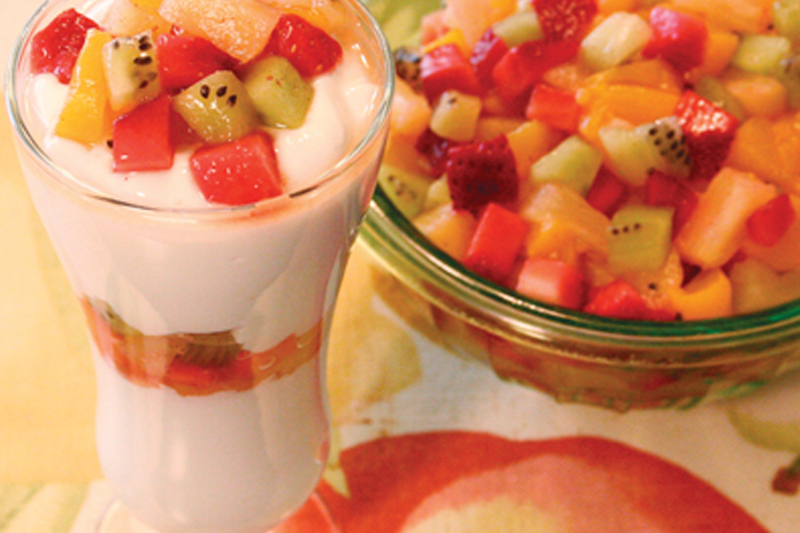In this vibrant photograph, the focal point is a tall, hourglass-shaped glass on the left, filled with an enticing fruit parfait. The parfait features layers of diced fruit—kiwi, watermelon, strawberries, pineapple, and possibly peaches and oranges—resting on top, followed by alternating strata of creamy white yogurt and more mixed fruit down to the bottom. To the right, there's a glass bowl brimming with a colorful medley of chopped fruit, showcasing chunks of strawberry, kiwi, cantaloupe, watermelon, and perhaps orange or grapefruit slices. Both the parfait and the fruit salad are situated on a floral tablecloth, predominantly white with splashes of red, yellow, and green hues suggesting flower petals and fruit shapes, adding to the overall freshness and appeal of the setting.